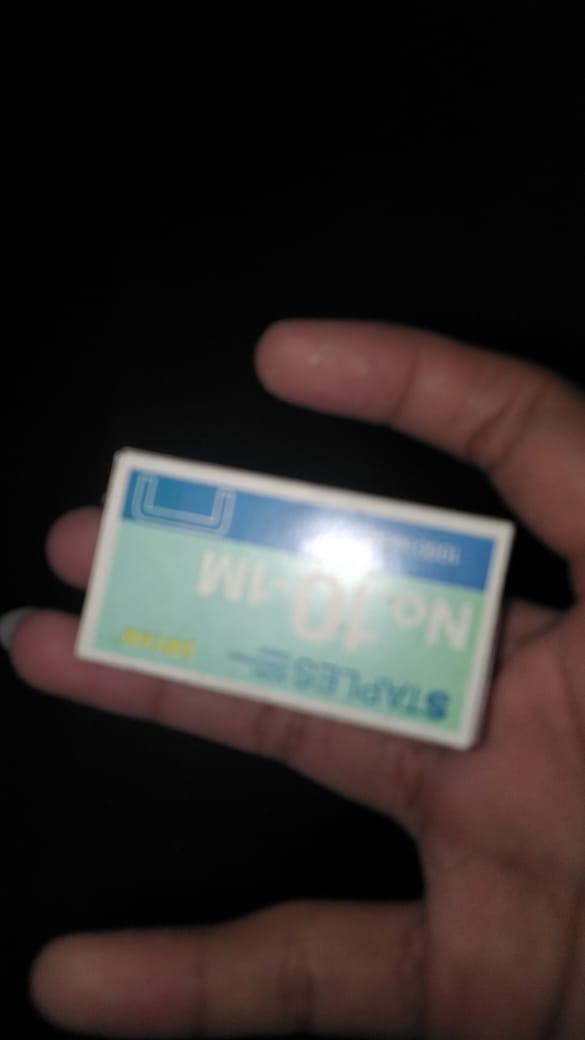In a low-quality, blurry photograph set against a pitch-black background, a person's right hand is shown, with the product resting on their ring and middle fingers. The product is a slim, rectangular cardboard box of staples, identifiable by its white border and text despite the blur. The box, which features light greenish or turquoise hues, is held upside down, making the text difficult to read. However, the readable text includes "number 10 1M." The image is focused solely on the hand and the staple box, with no other elements present.